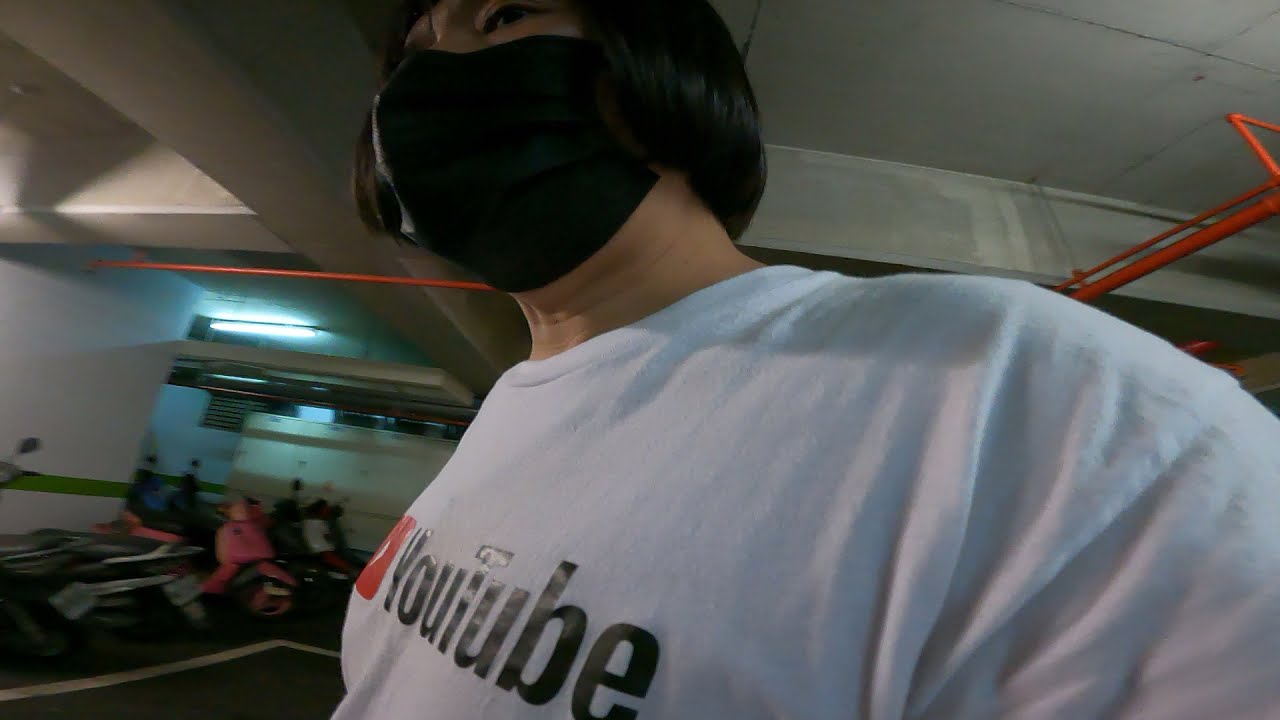In this wide rectangular image, we observe a person with light skin, identifiable as male, donning a white t-shirt that prominently displays the YouTube logo in bold, shiny black letters and a red symbol. His short, black hair peeks out from above a large black face mask that covers the lower half of his face. The person's shoulder dominates the bottom right corner of the image, with part of the chest and t-shirt visible. 

Above the person, the gray, geometric, and uneven ceiling is punctuated by red pipes and poles, likely part of a fire safety system. To the left, an indoor parking area is visible, featuring several scooters, or possibly mopeds, lined up in a row. The background hints at an industrial or functional space, maybe a parking garage or a similar structure. The room's ambiance suggests a utilitarian setting, characterized by the cement ceiling and the array of red piping.